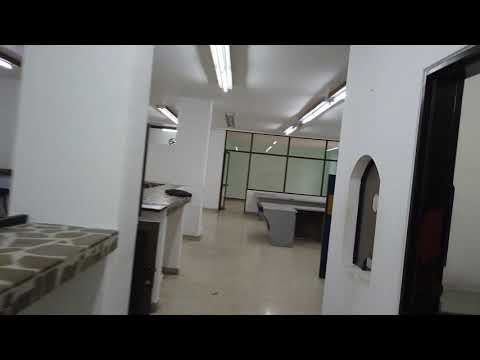The photograph captures an empty room inside a building, possibly a showroom or office space, characterized by its prominent white walls and ceilings adorned with long fluorescent tube lighting. The room features a foreground with a gray, stone countertop with thick white grout to the left, framed by a white pillar. To the right, closer to the image's front, is a doorway with a black frame and a window adjacent to it, possibly for communication, though it is closed and opaque. Moving deeper into the room, another white pillar is visible alongside various empty tables or countertops, which vary in appearance—some resembling stainless steel with white bases. The flooring appears to be light tan or white tile or linoleum. Toward the back of the room, a large gray table is situated not far from a glass wall with a black frame, obscured by tinted glass that light enters through, emphasizing the room's spacious, open-plan layout.